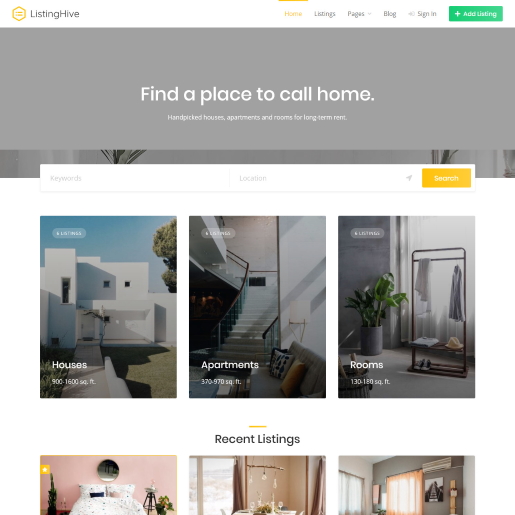The image is a detailed screenshot of the homepage of a website named "Listing Hive." Positioned at the top-left corner, the website name and logo are prominently displayed. On the top-right, the menu bar is visible with multiple options: Listings, Pages, Blog, Sign In, and a distinctive, large green button labeled "Add Listing." The "Sign In" option is highlighted in yellow.

Dominating the homepage is a welcoming headline that reads, "Find a Place to Call Home," accompanied by a smaller, unreadable sentence underneath. Below the headline, a large search bar is presented, allowing users to enter keywords and specify the location before clicking the "Search" button to view corresponding listings.

Further down, the homepage features three square sections each representing different types of properties users can search for: houses, apartments, and rooms. Each section includes a representative image.

The bottom part of the screenshot hints at an additional section titled "Recent Listings." This partially visible section displays three more square segments, presumably representing recent property listings or categories similar to the previously shown houses, apartments, and rooms. The content of these segments is largely cut off due to the screenshot's limited view, suggesting that a full view would reveal more information if scrolled down.